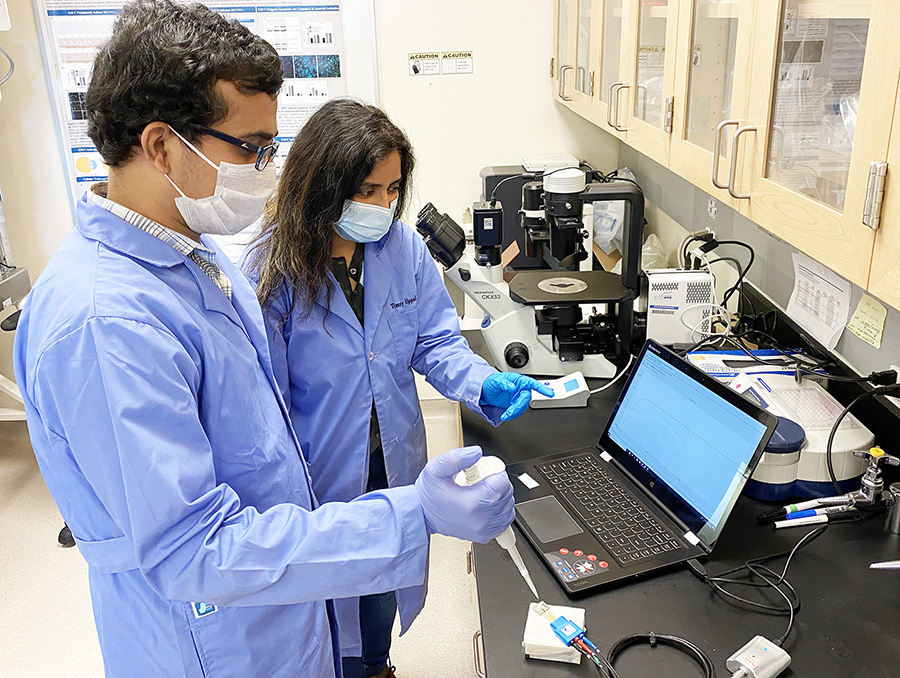In the photograph, a young man and woman, likely doctors or scientists, are diligently working in a laboratory setting. They are both dressed in blue lab coats and blue rubber gloves, and they wear white masks over their faces. The man, with brown hair and glasses, holds a syringe in one hand, which he appears to be using to deposit liquid onto a white square on the black table or countertop in front of him. The woman, with long brown hair, also wears a mask and gazes intently at the screen of a black laptop that rests on the table. Both are engaged in pointing at something on the laptop screen, suggesting a collaborative effort in their work. Surrounding them are various pieces of lab equipment, including microscopes, and you can spot a backdrop of white and black colors dominated by a black table surface. Cabinets with glass fronts, filled with additional lab equipment, line the wall behind them, alongside images of lab results, enhancing the scientific atmosphere of the scene.